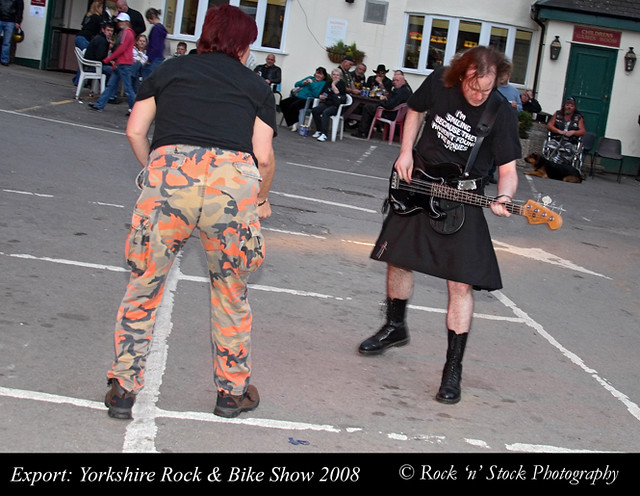In this rectangular, daytime photograph, captured at the Export Yorkshire Rock and Bike Show 2008 and credited to Rock and Stock Photography, two men are central to the scene, performing in a parking lot with a lively crowd in the background. On the right, a musician of Caucasian descent is playing a black electric guitar. He has long, straight brown hair that is thinning at the top and is dressed in a black short-sleeved T-shirt with an indistinct white print, a black kilt, and black boots. To his left stands another person, facing away from us, with dyed red shoulder-length hair. This individual is clad in a short-sleeved black T-shirt and camouflage pants featuring hues of orange, black, yellow, and gray, seemingly engrossed in the performance. The scene unfolds on a patchwork grey cement paved area adjacent to a tan stucco building with numerous white-framed windows and a green door. A crowd seated on white plastic chairs, along with a dog, can be seen enjoying the show, contributing to the dynamic and vibrant atmosphere of the event.